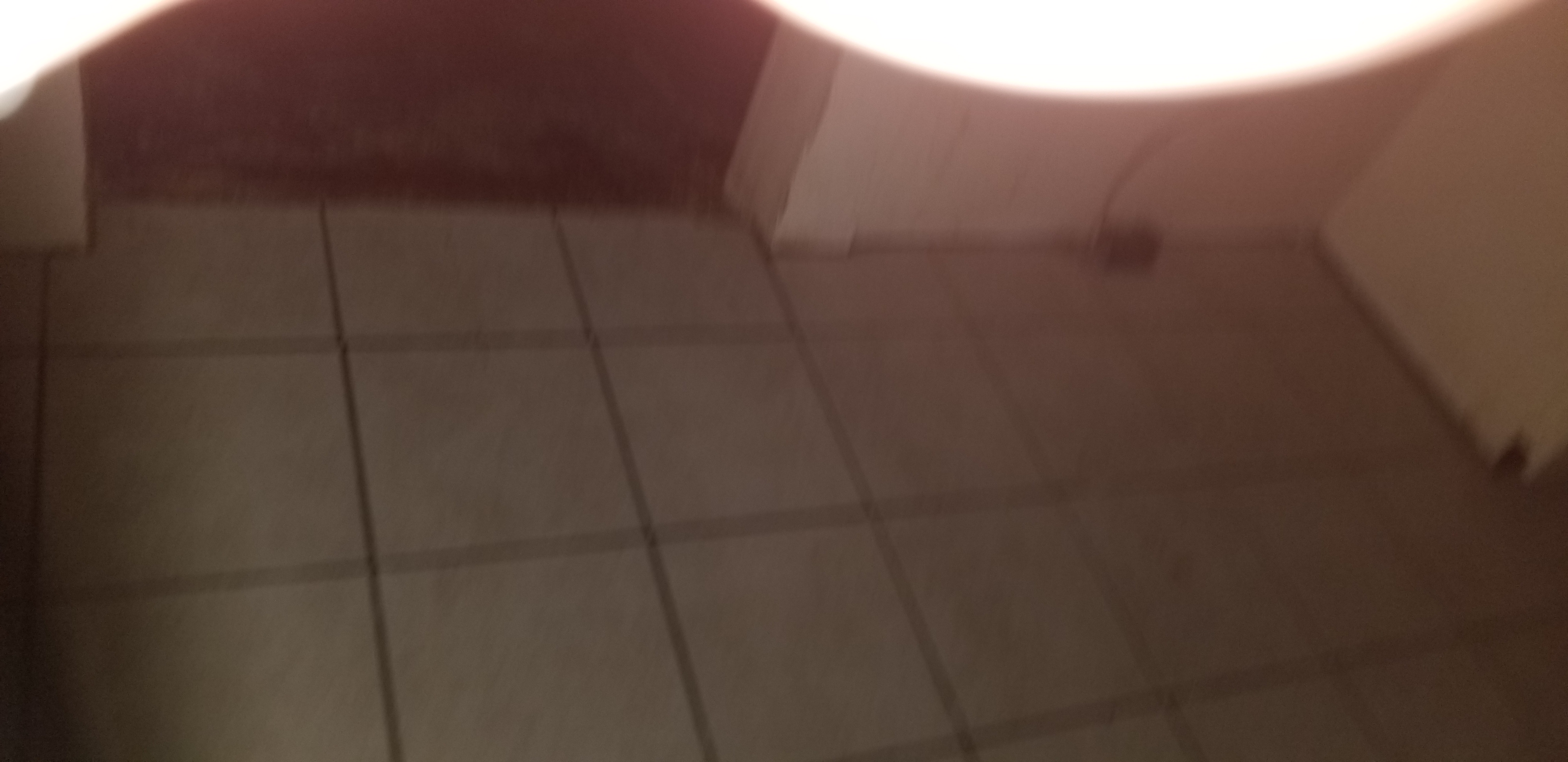The photograph, though blurry and panoramic in orientation, captures the corner of a room. The flooring consists of large, white square tiles, separated by gray grout lines. A white wall is visible in the corner of the room, enhancing the starkness of the tiles. In the upper left corner, there is a dark, pitch-black area, possibly an open door leading to the outside at night, though its exact nature is ambiguous. In the upper right portion of the image, a peculiar black square with an indistinct line extending from it further adds to the enigma of the scene. Additionally, the upper left corner is illuminated by an intensely bright light, perhaps emanating from a lamp, which adds a sharp contrast to the otherwise muted tones of the room. The overall blurriness of the photograph makes it difficult to derive clear context from the elements depicted.